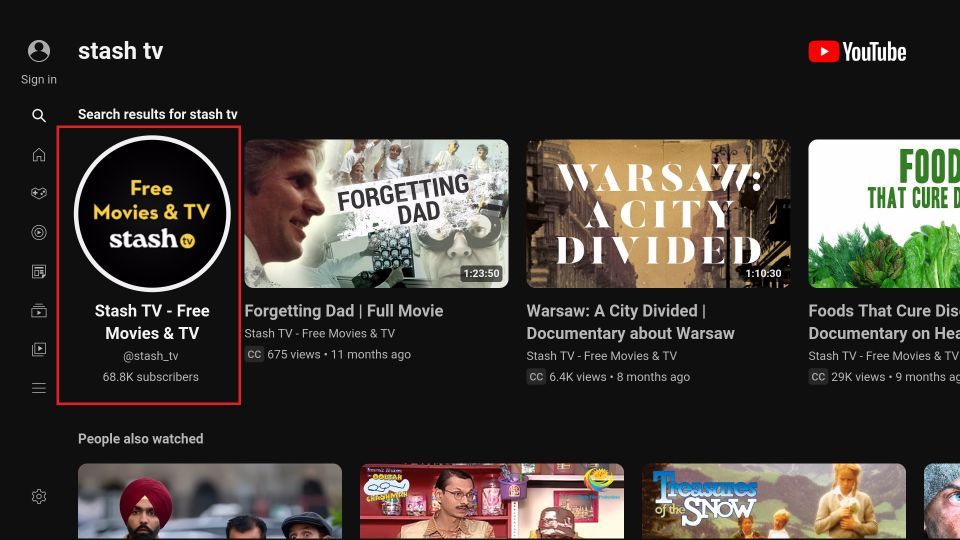This is a screenshot of a YouTube web page, prominently displaying the YouTube logo and name in the top right corner. On the left side, the text "Stash TV" is visible in white lettering. There is a sign-in option, below which are several icons including a search icon, a homepage icon, a heart or favorites icon, and a settings icon. 

A large red rectangular banner dominates the screen, bearing the text "Free Movies and TV, Stash TV, Stash TV, Free Movies and TV" alongside a subscriber count of 68.8 thousand. Below this banner, the featured movies include "Forgetting Dad, Full Movie" with an accompanying screen grab from the film. Another feature is a documentary titled "Warsaw, A City Divided," and a third movie shown partially is "Food That Cures DIS," which appears to be another documentary from Stash TV.

Towards the bottom of the screenshot, under the heading "People Also Watched," there are several partially displayed images of movies that viewers had also watched. Only one of these titles, "Treasures of the Snow," is fully legible.